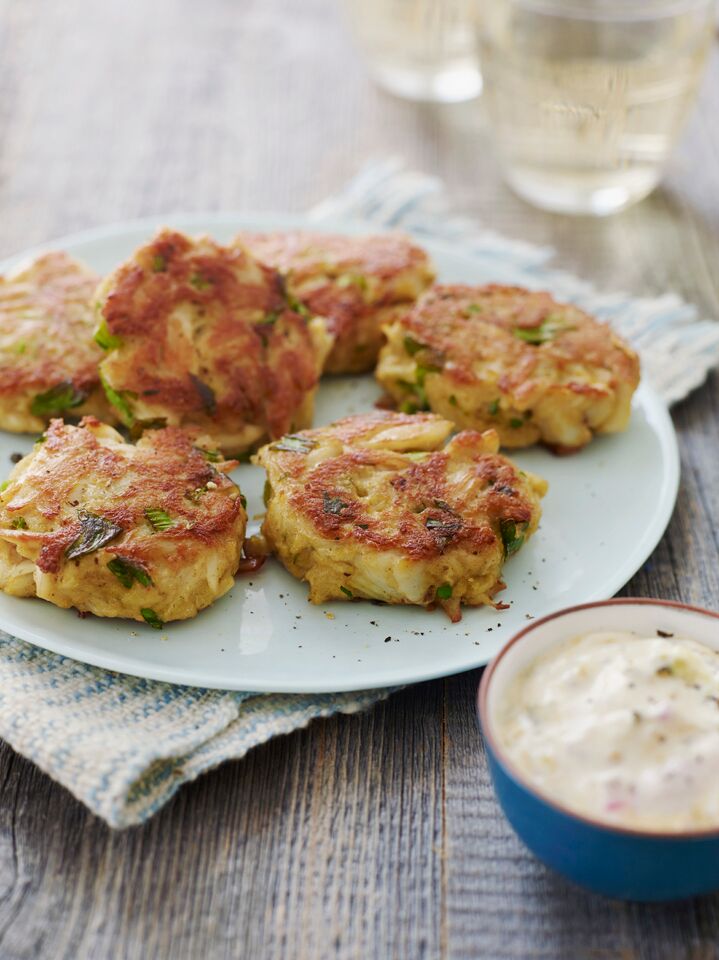In this culinary photograph, a white round plate showcasing six golden-brown crab cakes, seasoned to perfection with a crusty exterior, is the star. The plate rests on a folded, blue and white-striped linen napkin placed on a wooden surface with varied hues of grays, tans, and browns. Nestled next to the crab cakes is a small blue bowl of creamy tartar sauce. The scene also features two clear glasses of light golden beverage positioned further back on the surface, adding an elegant touch to the spread. Scattered around the plate are a few crumbs, emphasizing the freshly baked appeal of the crab cakes. The entire setup exudes a rustic yet refined aesthetic, perfect for a delectable dining experience.